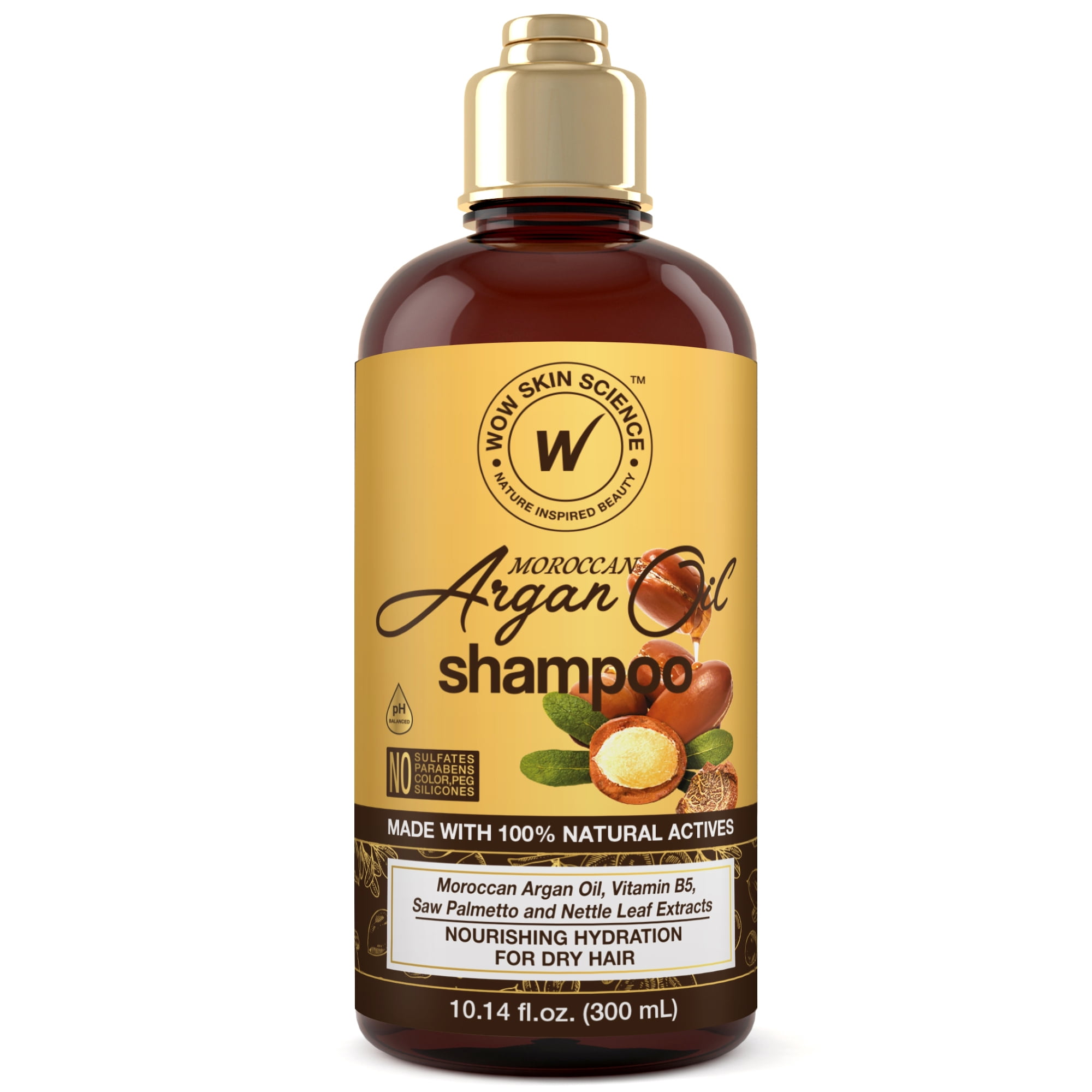The image displays a brown, semi-translucent bottle of shampoo against a white background, suggesting it's a product for sale, like on an online marketplace such as eBay. The bottle features a distinctive gold cap and a yellow label with a golden and brown color scheme. At the top of the label, the brand "Wow Skin Science" is prominently displayed alongside the slogan "Nature Inspired Beauty" within a circular design. Below, the label reads "Moroccan Argan Oil Shampoo" and highlights key ingredients: Moroccan argan oil, vitamin B5, saw palmetto, and nettle leaf extracts. It emphasizes the shampoo’s benefits for dry hair, stating it provides nourishing hydration. The bottle contains 10.14 fluid ounces (300 ml) and is marked with claims such as "Made with 100% natural actives" and free from sulfates, parabens, color Peg, and silicones. The label also features an image of Moroccan argan nuts and green leaves, reinforcing the natural theme.